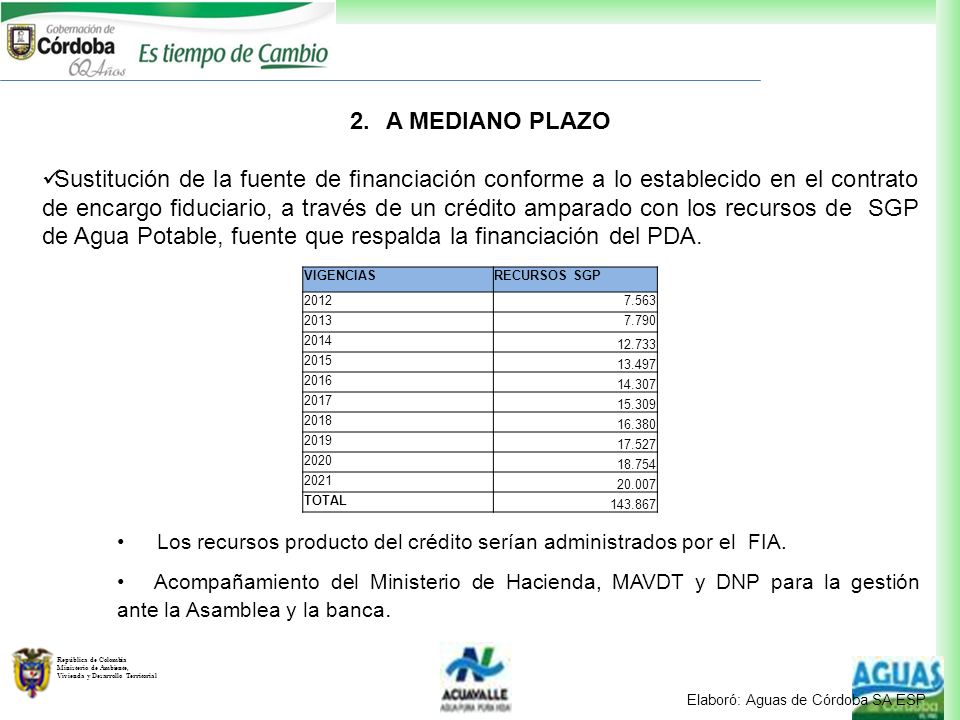The image, set against a white background, features a green border on the top and right side, transitioning from dark green on the left to light green. In the upper left corner, the text "Gobernación de Córdoba" is displayed in black, followed by "Estiempo de Cambio." Below this, centered in the image, it reads "02 Años, Mediano Plazo" in black letters. Beneath this header, there is a three-line paragraph in Spanish, which cannot be read clearly. A chart sits below the paragraph, divided into two main columns with approximately ten rows. The left column labeled "Vigencias" lists years from 2012 to 2021, and the right column labeled "Recursos SGP" lists corresponding numerical values with decimals for each year. The annual values in the chart are 7.563 for 2012, 7.790 for 2013, 12.733 for 2014, 13.497 for 2015, 14.307 for 2016, 15.309 for 2017, 16.380 for 2018, 17.527 for 2019, 18.754 for 2020, and 20.007 for 2021. The total value at the bottom of the chart is 143.867. In the lower right-hand corner of the image, the word "aguas" is written in blue letters.